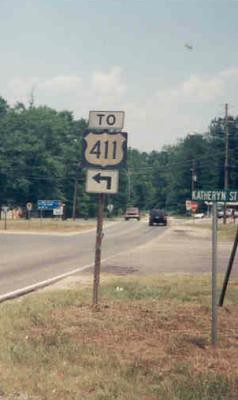A slightly blurry photograph taken on a sunny day, depicting a rural intersection on a country road. The grass visible in the scene is notably brown and dry, indicating dehydration or lack of maintenance. In the foreground, a two-lane road stretches horizontally, with a car traveling in each direction. At the corner of the intersection, there stands a green street sign with white lettering on a metal pole reading "Catherine Street." Adjacent to this, another metal pole supports a white rectangular sign with a black arrow pointing left, indicating a permissible left turn. Below this left-turn sign, a black state route marker displays the number "411" within a white shield design, and above it, a smaller white sign shows the number "2." In the background, a dense line of tall trees frames the road, which continues into the horizon, blending into the lush canopy.